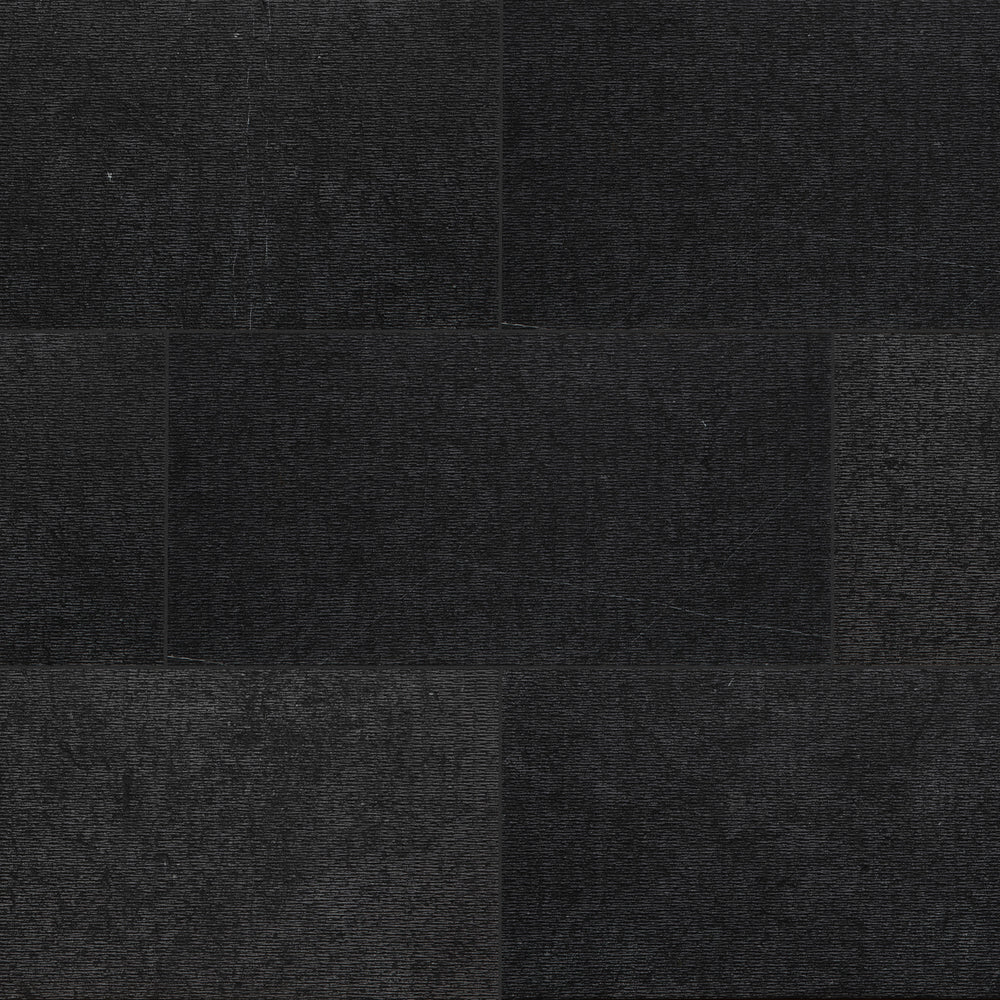The image depicts an arrangement of black rectangular and square blocks with varying shades, ranging from dark black to gray and charcoal. At the top, there are two equal-sized squares, one being the darkest black on the top right. The middle section features a vertical rectangle flanked by a horizontal rectangle and another vertical rectangle of the same size as the one on its left. At the bottom, the layout mirrors the top with two matching rectangles or squares, where the bottom left block appears slightly grayer than the others. The blocks seem to possess a tactile texture, with visible grains, scratches, and dust, and some even have slight pulls and catches, suggesting a material-like quality such as fabric or tile with a staggered brick or subway tile pattern. The overall feel is that of a scanned texture image, possibly used for overlaying in digital design or photoshopped images.